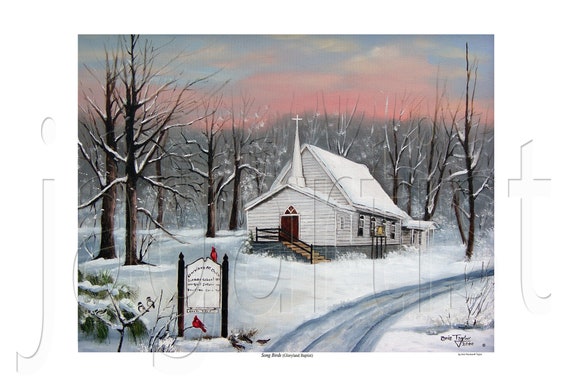In this picturesque winter scene, a quaint country church, painted white, stands amidst a snowy landscape. The church, complete with a steeple adorned by a cross, features a maroon door accessed by steps at the front. The roof, blanketed with snow, complements the overall serene atmosphere. Surrounding the church are leafless trees, their branches dusted with snow, enhancing the wintry charm.

The sky behind the church transitions from a soft pink near the horizon to a clear blue as it rises, scattered with white and pink clouds, suggesting either dawn or dusk. In the foreground, a small, winding road leads to a white sign at the entrance, on which two vibrant red male cardinals are perched—one on top and one on a lower branch.

Additional details include another door and several windows on the right side of the church, as well as various young trees and bushes within the vicinity, all covered in snow. This idyllic scene, reminiscent of a Christmas card, evokes a timeless, peaceful winter's day.